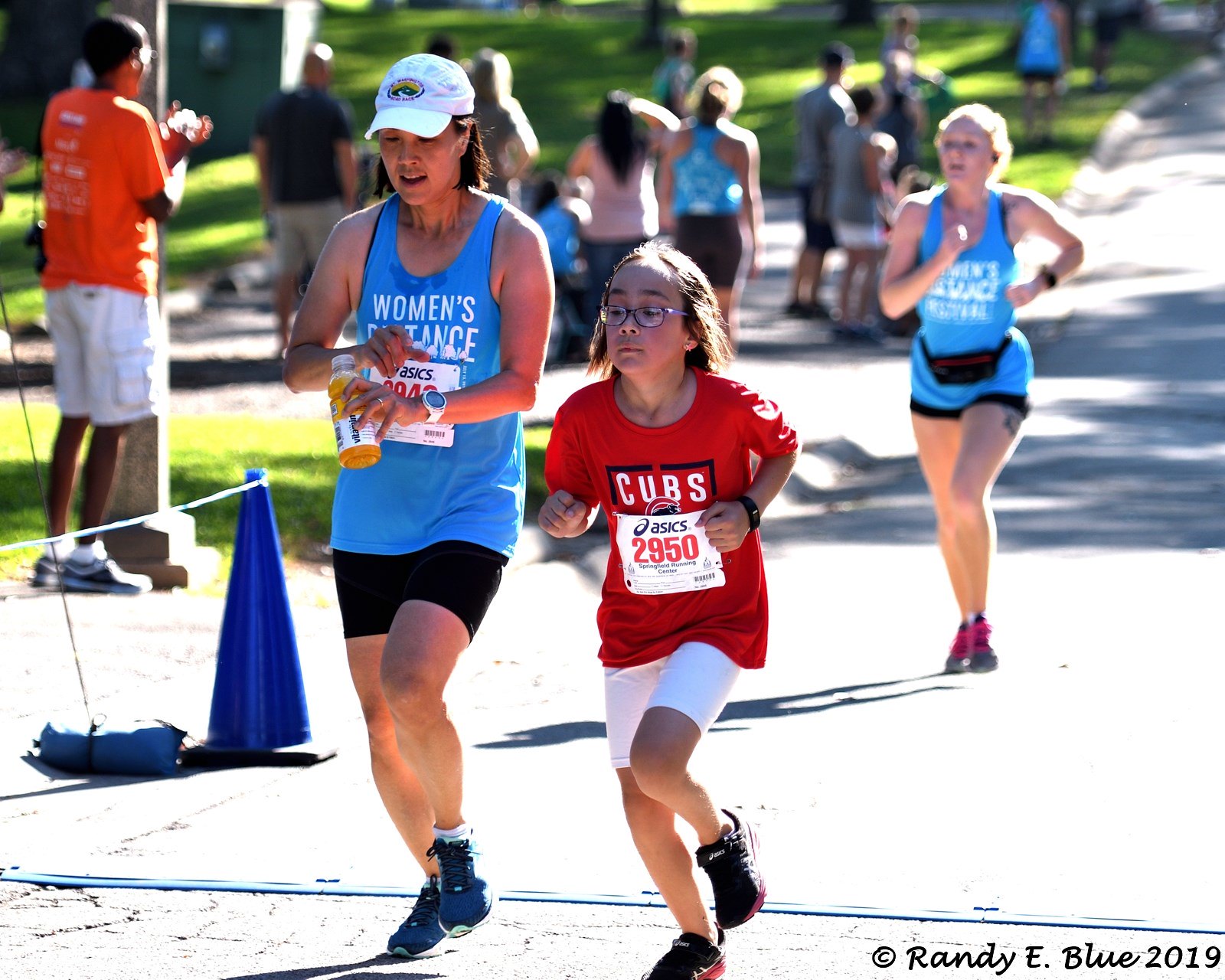The image captures a vibrant scene of a women's road race, marked by the shared enthusiasm of both participants and spectators. In the foreground, a nearly middle-aged woman, dressed in a light blue sleeveless t-shirt with the text "Women's" visible, runs at a slight angle. She's equipped with black shorts, black shoes, and a white cap with an emblem, while holding an orangey vitamin water in her left hand. Beside her is a young girl in a red Cubs shirt with white shorts and black sneakers, her race number "2950" prominently displayed on a white tag pinned to her shirt. Both runners exude determination as they propel forward. In the background, another woman in similar blue attire runs with her arms extended in motion. Spectators line the grass section to the left, one of whom is a man in an orange shirt, clapping in encouragement. The scene is set against a backdrop of concrete and grass, with the signature "Randy E. Blue 2019" marking the bottom right corner, attributing the photograph to its creator.